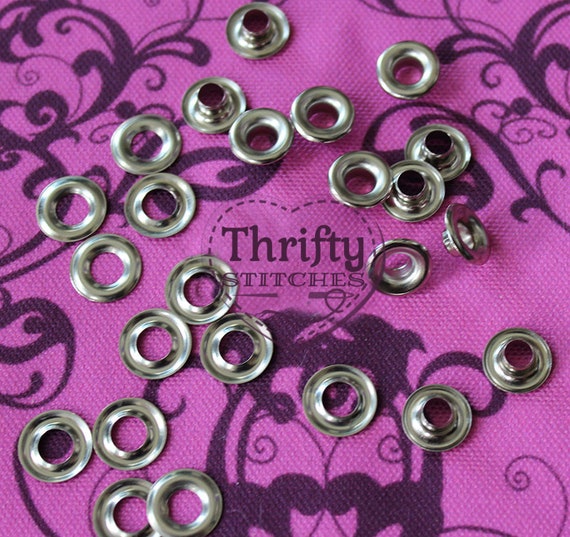In this detailed color photograph, a close-up view reveals an array of silver metal grommets scattered across a lavender purple fabric. The fabric, adorned with a decorative swirly pattern in varying shades of purple, serves as an intricate backdrop. At the center of the image, enclosed within a heart design adorned with a needle and stitching, lies the text "Thrifty Stitches." The grommets, appearing in two parts with some having an extended piece, are typically used to reinforce pre-cut holes in fabrics, such as those found in corsets, hoodies, or swim trunks. The scene is illuminated by natural daylight streaming from a window, likely positioned to the left, enhancing the details and colors of the composition.